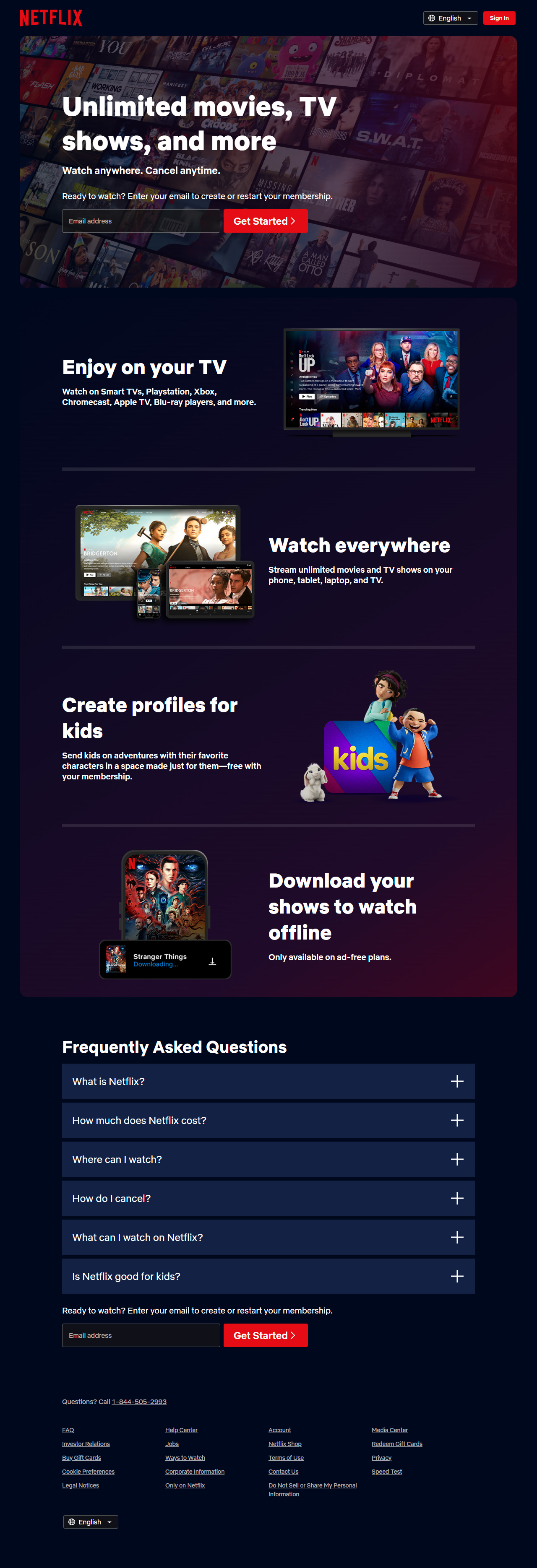The background of the image is a deep, dark blue, almost black. In the top left corner, a bright red "Netflix" logo stands out. On the opposite side, "English" is written in white text. Below this, a red box labeled "Dinah" appears prominently. Across the center of the image, various Netflix shows and movies are depicted, including titles like "The Cruise," "Missing," "A Man Called Otto," "SWAT," "Diplomat," "Shameless," "Flash," "Bad Guys," and "You."

Overlaying these visuals, a bold white text declares, "Unlimited Movies, TV Shows, and More. Watch anywhere, anytime. Ready to watch? Enter your email to create or restart your membership." 

Beneath this text, a white-outlined rectangle with the words "Email Address" written inside it invites users to input their information. Adjacent to it, a red box with white text prompts with "Get Started."

Further down, another section in white text explains the streaming capabilities: "Enjoy on your TV. Watch on smart TVs, PlayStation, Xbox, Chromecast, Apple TV, Blu-ray players, and more." On the right-hand side, it states, "Watch Everywhere. Stream moments from movies and TV shows on your phone, tablet, laptop, and TV."

To the left, a message encourages creating personalized profiles: "Create Profiles for Kids." On the right again, it highlights the flexibility of offline viewing: "Download your shows to watch offline."